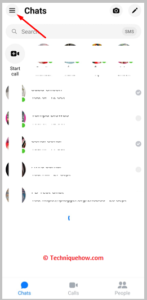This is a blurry screenshot of Facebook Messenger's interface. Despite the image quality, it is evident that the screenshot captures various elements of the popular messaging app. At the top left, the word "Chats" is visible, indicating that this is the chat overview screen. Just below the header, there are different profile icons representing the user's contacts. Each contact's name and profile picture are obscured by white lines, presumably for privacy reasons.

The bottom portion of the image displays a list of conversations. Next to each conversation, there are indicators showing whether the messages have been seen or if the contact is currently online. Most of these conversations feature a gray checkmark to the right, suggesting that the recent messages have not been read by the recipients.

At the top of the screen, there is a search bar for quickly finding contacts without scrolling through the entire list. Additionally, on the right side of the search bar, there are icons for starting a video chat, taking a picture, and a pen icon likely used for composing or editing messages. Despite the blur, the layout and functionality of Facebook Messenger are recognizable.